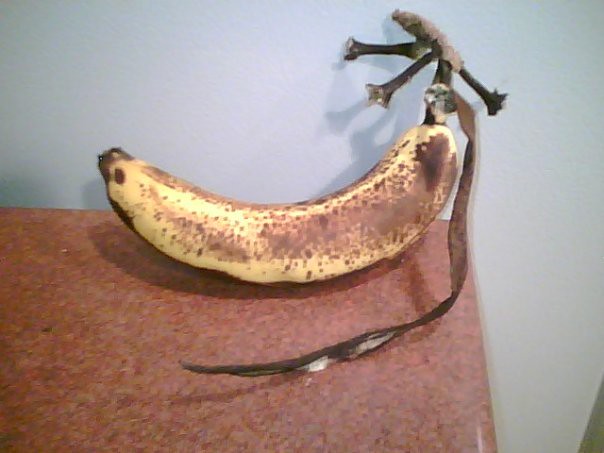The photograph depicts a single overripe banana, the last remaining one from a bunch. It is positioned precariously on the edge of a speckled red and grey counter, which features a rounded edge and is set against a white wall that appears slightly grey due to the lighting. The light source is above and to the right, casting a distinct shadow of the banana onto the wall. The banana is part of a bunch originally containing five, evidenced by the main stalk and four where previous bananas were detached. An additional detail shows that when one of the bananas was removed, a strip of its peel was left hanging from the stalk, now blackened and twisted. The banana itself retains some of its yellow hue, but is predominantly covered in brown spots, indicating its advanced ripeness and potential bruising. It leans against the wall, with its curved end resting on the counter.